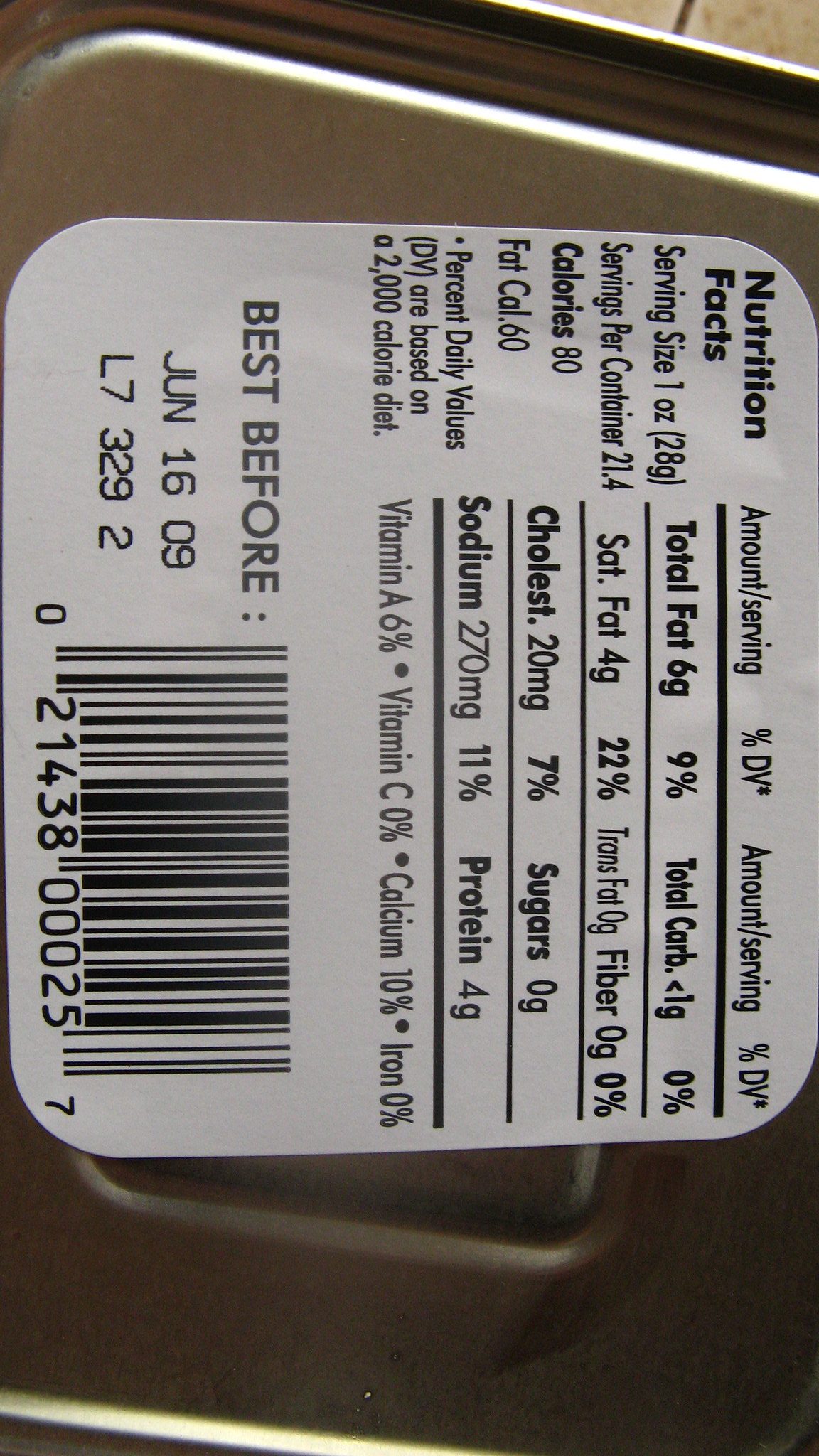The image depicts the back of a silver-colored can, possibly a food or beverage item. The can features a nutrition facts label detailing various components: it indicates the serving size as one ounce with a total fat content of 9 grams. Additionally, the label lists 278 milligrams of sodium. Interestingly, there are no visible ingredients listed alongside the nutrition information. The can also has an expiration date, marked as "Best before June 16, 09," suggesting that the can is quite old. Despite the nutritional data, other identifying information about the can's contents is absent.